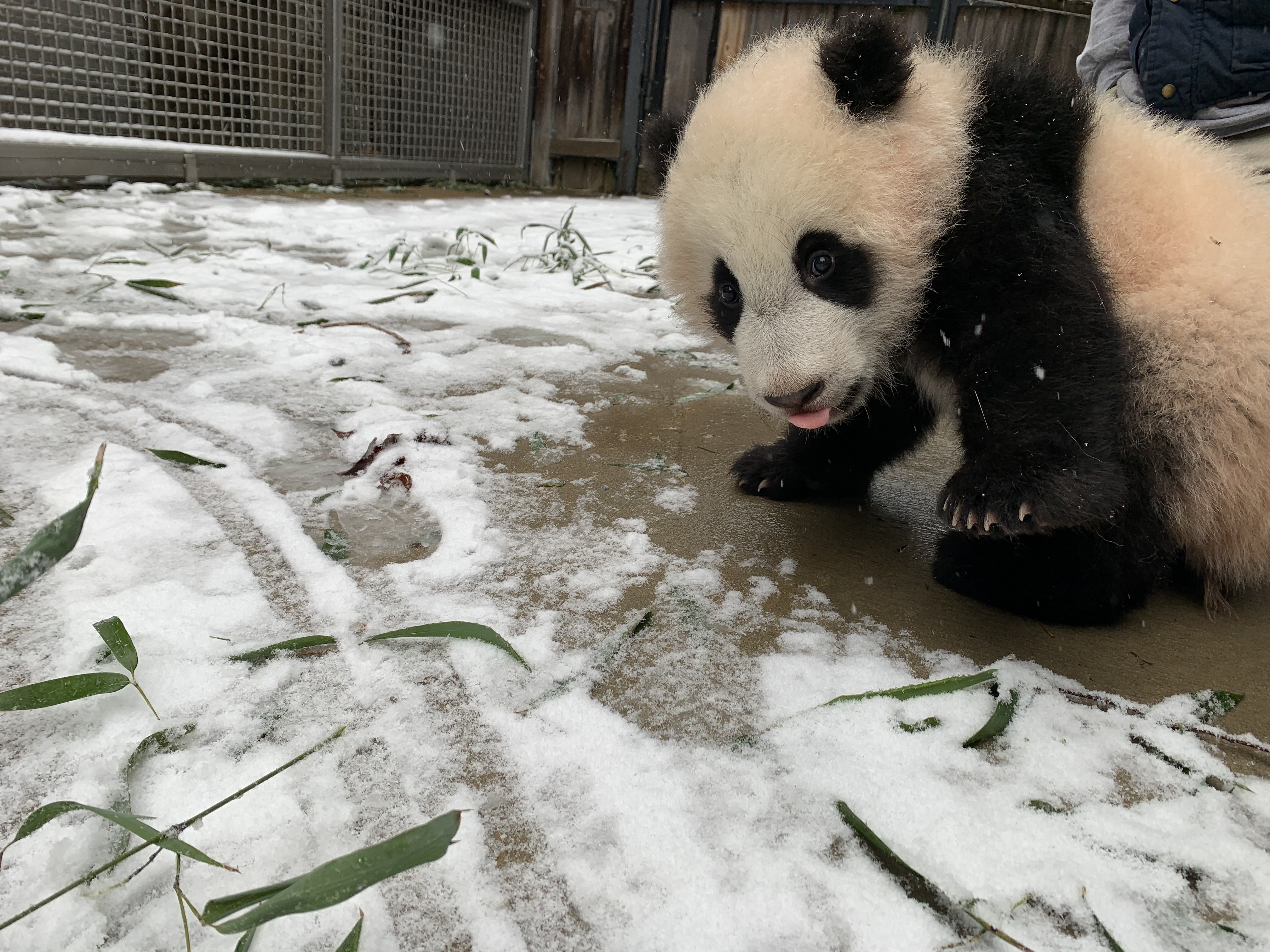A baby panda bear with distinct black and white fur is captured in a snowy setting. Positioned on the right side of the scene, the panda bear is resting on a snow-covered patch of ground interspersed with green bamboo leaves. Its tongue playfully sticks out as it gazes towards the left, adding an adorable touch to the image. Nearby, the sharp nails on its feet are visible. In the background, a brown slat fence and gate are partially visible, suggesting the setting might be a zoo. A person, possibly a caretaker in a jacket, stands beside the panda, also on the right. The overall atmosphere blends the natural beauty of the snow and bamboo with the structured elements of a zoo enclosure.